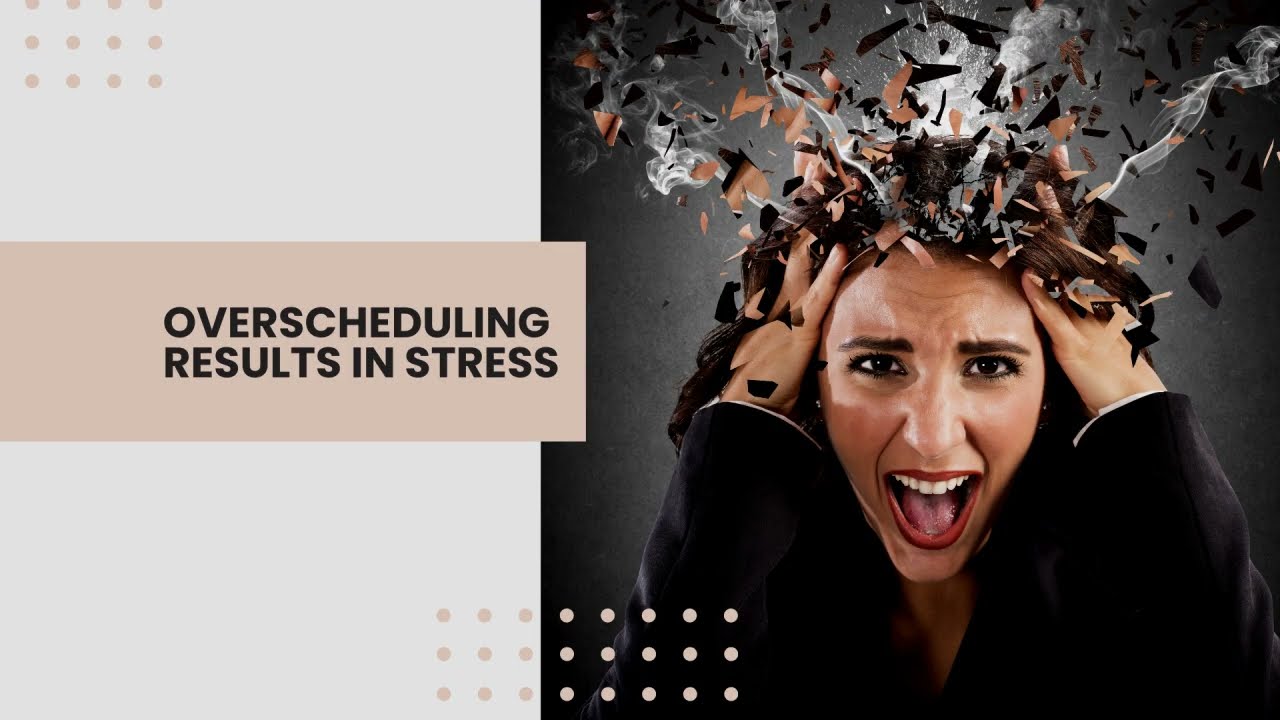The image is a horizontally oriented rectangle divided into two sections. On the left section, there is a gray vertical rectangle adorned with beige and gray dots. A horizontal beige bar in the center displays the text "Overscheduling results in stress" in black letters. The right section, taking up about 60% of the image, features a square photograph of a white woman framed from the chest up. She is wearing a long black jacket or sweater and has dark hair. Her expression is one of surprise or stress, with her mouth open as if she is screaming. Both of her hands are positioned at the sides of her head, giving the impression that confetti or animated particles are explosively emerging from her head, visually emphasizing her overwhelmed state. The overall design appears reminiscent of a work presentation slide or a guide for employees.